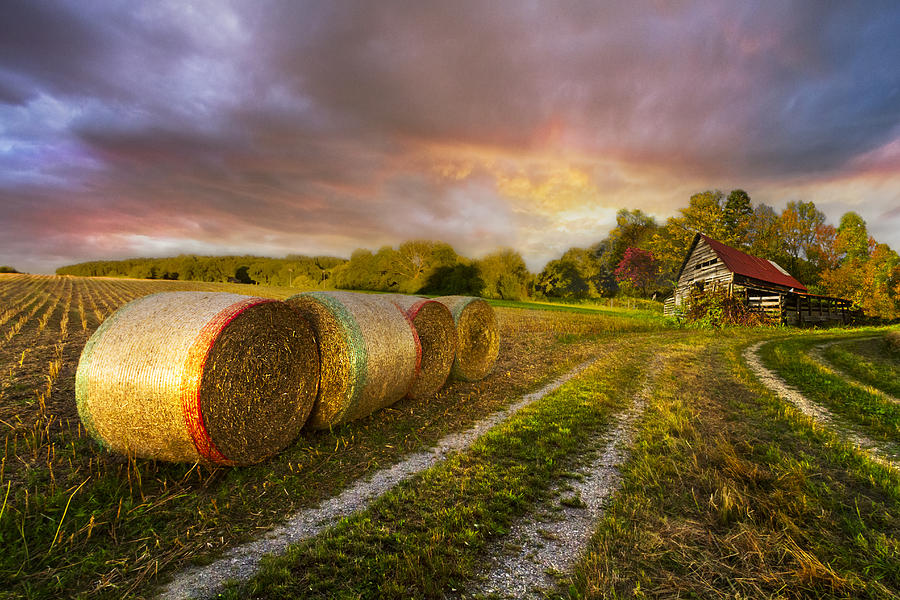The image depicts a picturesque farm scene that might have been computer-enhanced for vibrancy. In the foreground, four round bales of hay with green and red borders are neatly arranged in a grassy area. A gravel track, likely used by tractors or other vehicles, cuts through the landscape. To the right and slightly in the center stands an old, rustic wooden storage building with a red slanted roof, potentially a farmhouse or barn. This structure shows signs of wear, blending naturally with the setting. Behind the building and further into the background are a variety of trees displaying autumnal hues, suggesting the scene might be captured in late fall. Rolling hills and additional patches of farmland stretch into the horizon, where short waves of grain or possibly wheat are growing. The sky suggests an impending sunset, with partly cloudy skies painted in shades of yellow, white, light blue, purple, lavender, green, silver, and orange. The upper part of the sky is dominated by more ominous gray clouds, contrasting with the brilliant yellows and reds closer to the horizon. The absence of people and animals adds a serene, tranquil quality to the idyllic farm landscape.